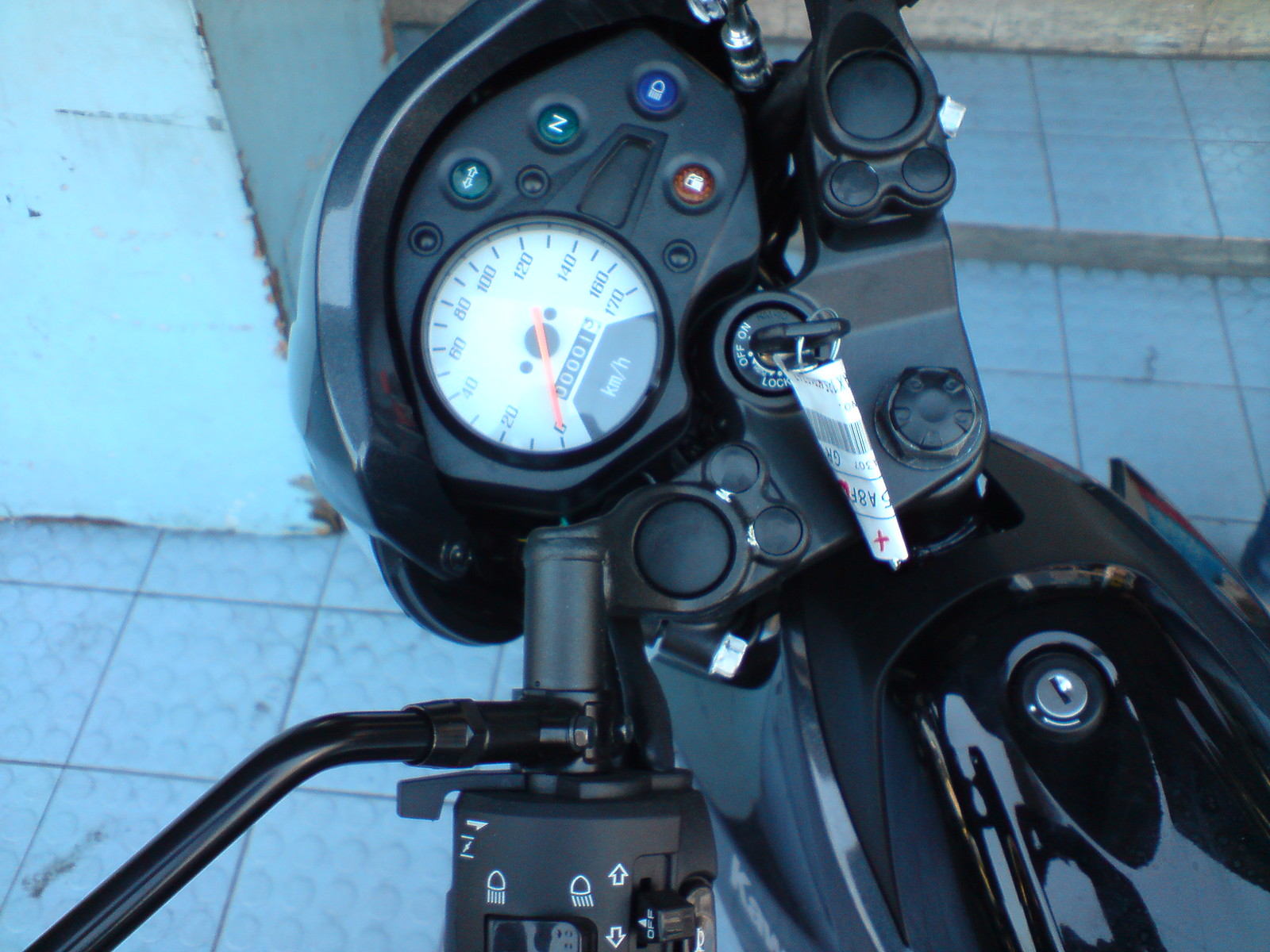A close-up of a motorcycle's front interface, providing the driver's perspective from the seat. Central to the image is the ignition with the key inserted, adorned with a small sticker. The speedometer, calibrated in kilometers per hour, ranges from 0 to 170. The dashboard features an array of multi-colored buttons: two green ones, one marked with an arrow for turning signals and the other with an "N" for neutral, a blue button with a white padlock symbol, and an orange button resembling a gas pump, likely for accessing the fuel compartment. The left handlebar is visible, angled downwards, revealing controls for adjusting the front light. The motorcycle's sleek black body is partially seen, including a secondary keyhole, potentially for the fuel compartment.